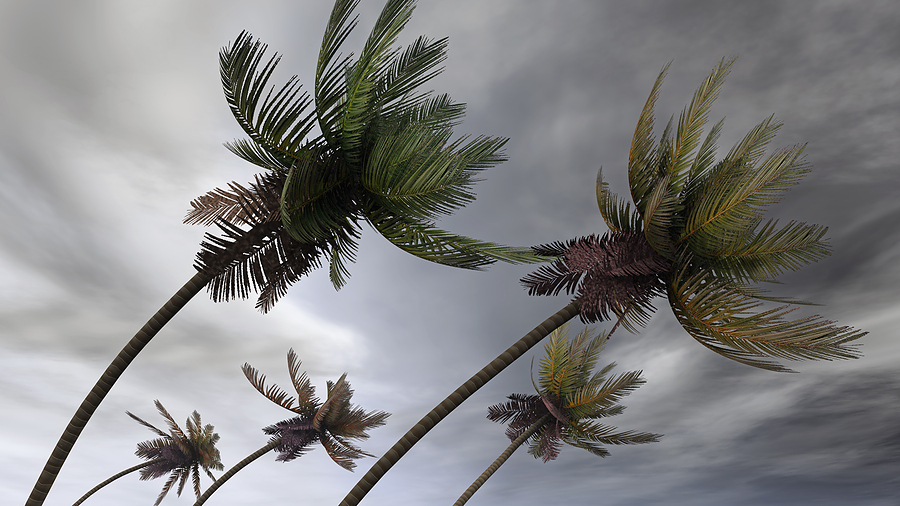Amidst a raging tempest, a row of five palm trees sways violently to the right, their trunks nearly bent at a 45-degree angle under the immense wind pressure. The two larger trees in the front and three smaller ones in the back all share the same fate, their green and yellowing leaves forced upwards against the torrent, some appearing ready to be torn away. The backdrop is dominated by a tumultuous sky, transitioning from dark, angry gray on the left, riddled with almost black patches, to a slightly lighter yet still foreboding gray on the right. Thick, swirling clouds engulf the entire scene, leaving no trace of blue sky, intensifying the sense of an impending hurricane.